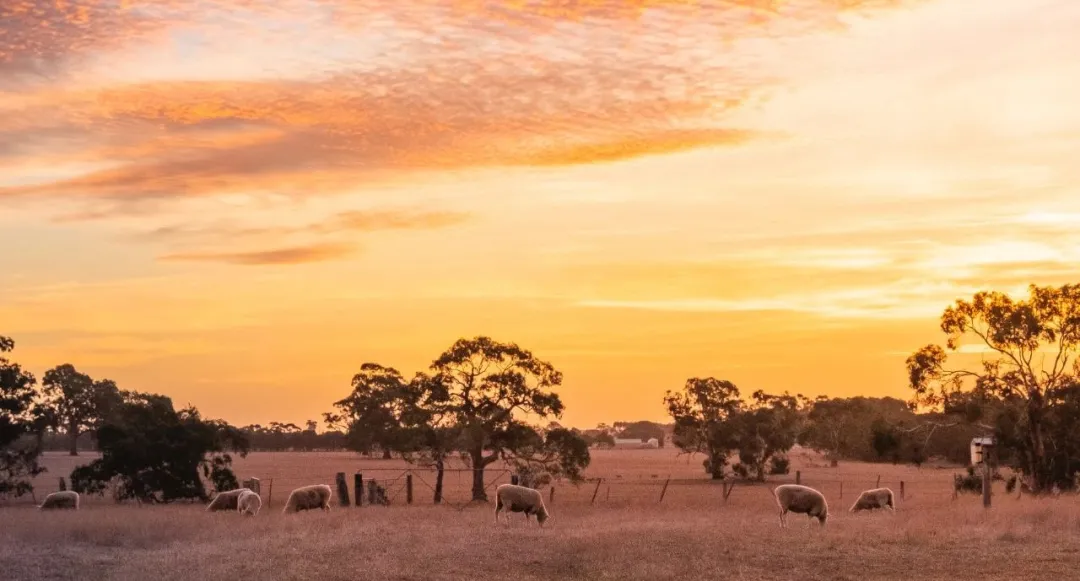The image captures a serene nature scene at either sunset or sunrise, characterized by an expansive field of grass where approximately eight sheep graze peacefully with their heads down. Scattered throughout the field are several large, old trees with massive trunks, and in the distance, a fence encloses the sheep, hinting at a remote farmhouse far off in the horizon. The sky, taking up roughly 75% of the frame, displays a stunning gradient of cream, light orange, pink, and gold hues, casting a warm glow over the grayish-brown meadow. The photograph is in landscape orientation, devoid of any text, and beautifully highlights the harmonious coexistence of wildlife and nature.